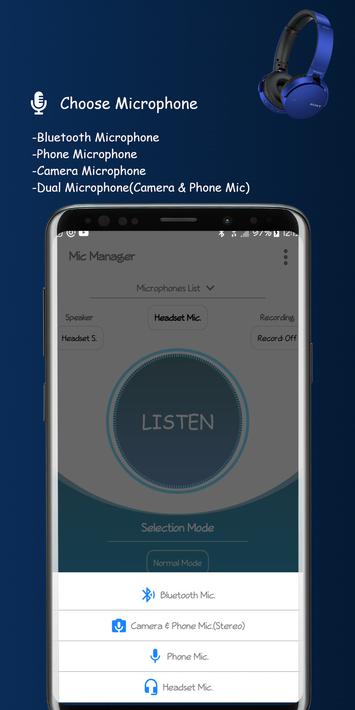A detailed screenshot features a dark blue border that extends from the top down about a third of the way and then continues down the right and left sides, approximately an inch wide. In the top-right corner, a pair of headphones is depicted: the left earcup shows the inside, colored black, while the right earcup shows the outside, colored blue. Below the headphones, a white microphone icon is accompanied by the text "Choose Microphone" in white. A list follows with options separated by dashes: "Bluetooth Microphone," "Phone Microphone," "Camera Microphone," and "Dual Microphone (Camera and Phone Mic)."

In the lower left section of the screenshot, an outlined phone with a gray border and white side borders is visible. The top of the phone screen shows standard icons in white for battery, time, and Wi-Fi. Below these icons, a faded gray popup tab occupies about two-thirds of the screen, transitioning to light blue. At the center of this section is a large light blue button labeled "Listen" in white.

Above this button, there is a white tab with "Handset Mic" written in black and a tab to the left labeled "Headset S," also in black. Further above lies the word "Speaker," while to the right is "Recording" and "Record Off." Near the top of this tabbed section is the term "Microphone List."

Underneath the blue "Listen" button, within the blue border, the phrase "Selection Mode" appears in white, followed by a white line and then "Normal Mode" encased in a white border. Below this area, the background turns white. Four sections list different microphone options with icons:

1. "Bluetooth Mic" with a blue Bluetooth icon.
2. "Camera and Phone Mic" with blue camera and microphone icons.
3. "Phone Mic" with a blue microphone icon.
4. "Headset Mic" with a blue headphone icon.